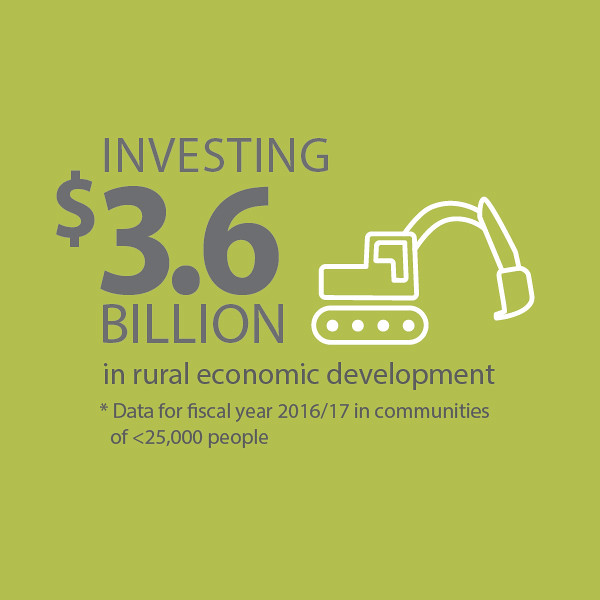The image is a large, solid green square with a vibrant olive or chartreuse background. In the center-left, bold dark gray text reads "INVESTING" followed by a large, block-style "3.6" with a dollar sign, beneath which "Billion" appears in similarly bold, uppercase letters. To the right of this central text, there is a minimalist white outline of a construction vehicle, likely a backhoe loader or excavator. Below the central text, further gray uppercase lettering states "IN RURAL ECONOMIC DEVELOPMENT." An asterisk-marked note is left-aligned at the bottom, detailing "Data for Fiscal Year 2016-17 in Communities of Less Than 25,000 People." The remaining lower part of the image continues the green background uninterrupted.